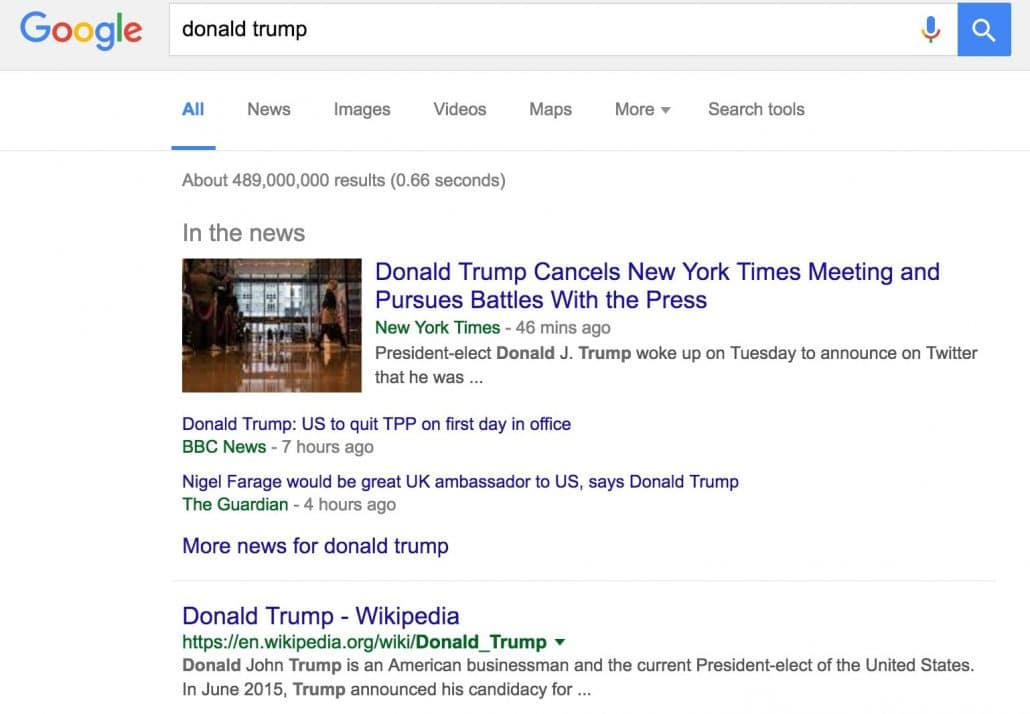This image is a screenshot of a Google search results page for "Donald Trump." At the top, it prominently displays the Google logo. Directly below is the search query "Donald Trump" with various categories such as All, News, Images, Videos, Maps, and More, along with search tools options. The search yielded approximately 489 million results in just 0.66 seconds.

Highlighted news articles include:
1. A New York Times headline from 46 minutes ago stating, "Donald Trump cancels New York Times meeting and pursues battles with the press," with a brief excerpt noting that President-elect Donald J. Trump announced this decision via Twitter.
2. A BBC News article from 7 hours ago reporting, "Donald Trump, U.S. to quit T.P.P. on first day in office."
3. A Guardian headline from 4 hours ago, "Nigel Farage would be great U.K. ambassador to U.S., says Donald Trump."

Additionally, there is a link to Donald Trump’s Wikipedia page with a brief summary mentioning that Donald John Trump is an American businessman and the President-elect of the United States as of the time of this search. 

The screenshot contains no images of people, animals, plants, trees, automobiles, helicopters, or airplanes.